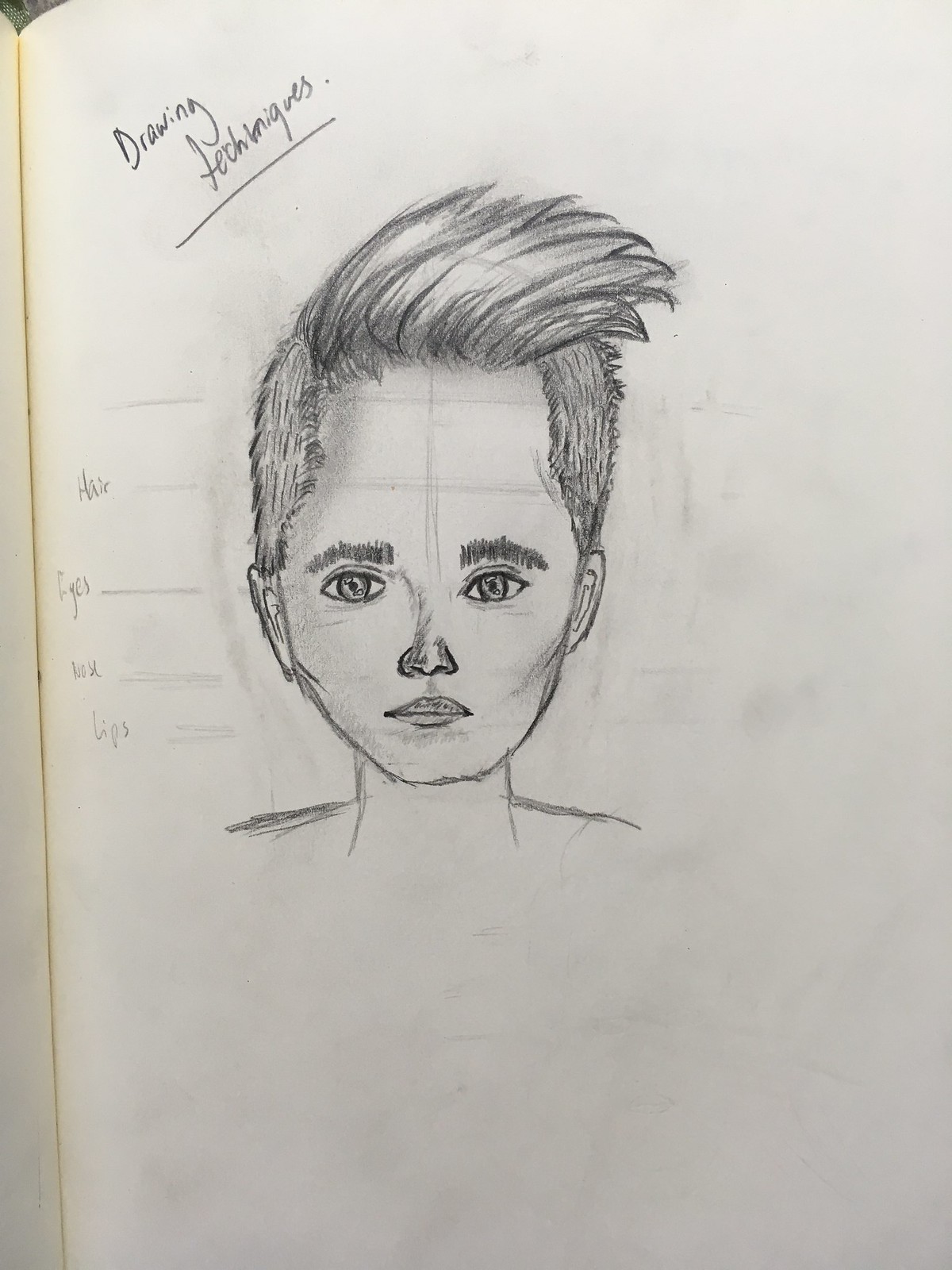The image depicts a pencil drawing on an off-white sheet of paper in a drawing notebook, evident from the visible spine on the left side. In the top left corner, underlined, is the label "Drawing Techniques." The central focus of the drawing is a detailed depiction of a man with a very prominent, broad forehead and short side hair, while the longer hair on top is styled to the right. His bushy eyebrows frame well-defined, centered eyes with eyelid lines. The figure's narrow nose and medium-sized lips are also meticulously sketched. The drawing extends to include the neck and shoulders, but not the rest of the body. Surrounding the head are annotation lines pointing to the hair, eyes, nose, and lips, and subtle smudge marks from erasing are visible throughout the page, indicating the artist's process.